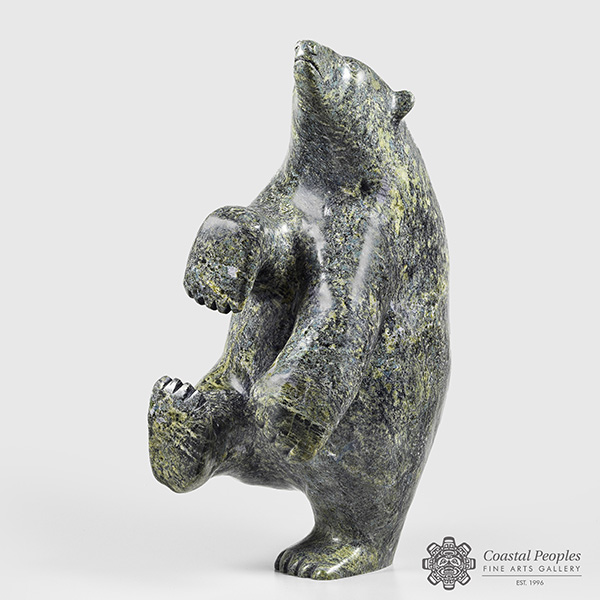The image captures a meticulously carved stone sculpture of a bear, gracefully balancing on its left rear paw while the right rear paw is extended forward. The bear's left front paw dangles downward, and its right front paw is slightly raised, creating a dynamic, almost mid-motion appearance. The bear's head is tilted upwards, as if observing something in the sky, possibly a passing plane, with its small, frowning mouth, visible nostrils, and ears subtly poking out at the sides. The sculpture’s texture boasts a polished, smooth surface, primarily black with intricate patterns of green and speckled bits of yellow, grey, and white. This detail suggests the stone is finely textured and enhances the visual depth of the piece. Situated in the bottom right-hand corner of the photograph is an inscription: "Coastal People's Fine Arts Gallery, established 1996," accompanied by a logo depicting a sun, indicating the sculpture's display location in the renowned gallery.